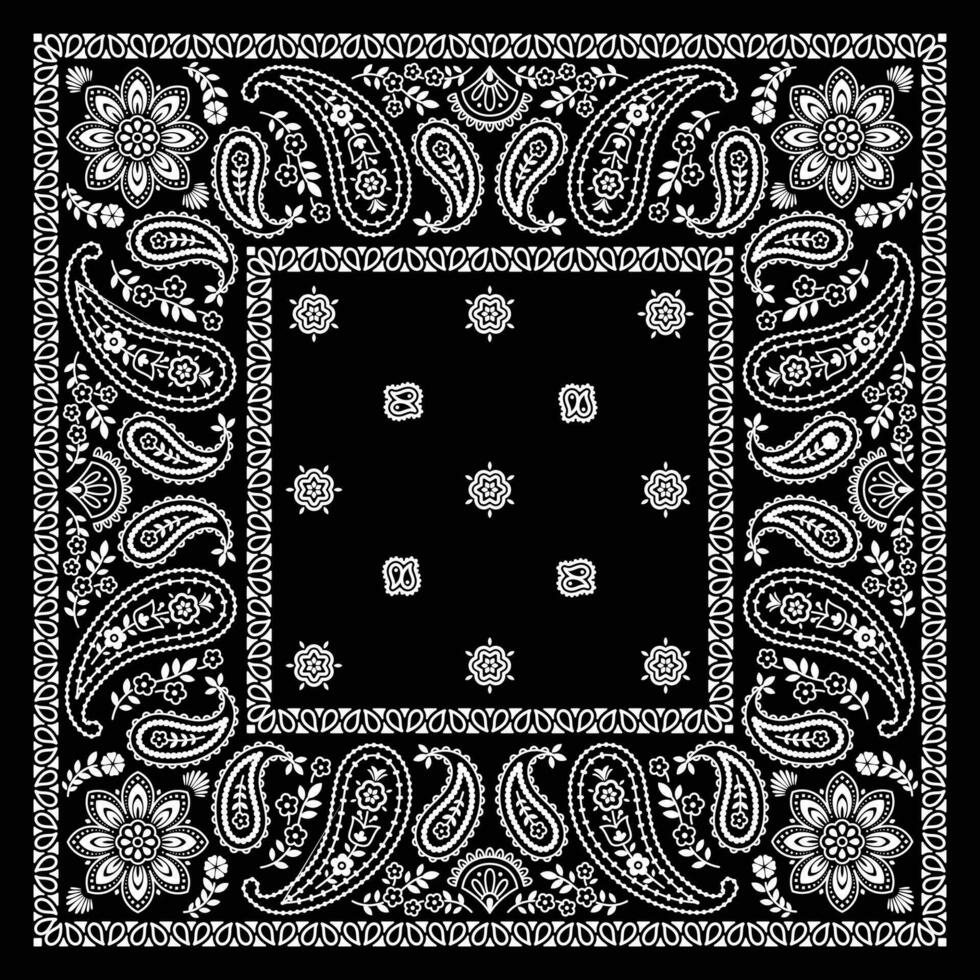The image depicts a highly detailed black and white bandana with an intricate paisley design. The bandana is fully spread out, occupying the entire frame and bordered by multiple layers. The outermost border is solid black, followed by a thin white and black border adorned with avocado-shaped motifs. Each corner features an eight-petaled flower, adding to the complex aesthetic. Inside this border is a larger section of black space punctuated by around 10 to 13 flower-like symbols, each unique and meticulously detailed, representing various floral and vegetative patterns. The inner area also contains another thin white and black border similar to the outer one, enhancing the overall symmetrical and repetitive but uniform design. This bandana could serve multiple purposes, such as a functional accessory for wiping sweat or as a representation of personal style, family, or crew. Its craftsmanship, whether a drawing, sketch, or photograph, emphasizes precision and elegance in its decorative elements.